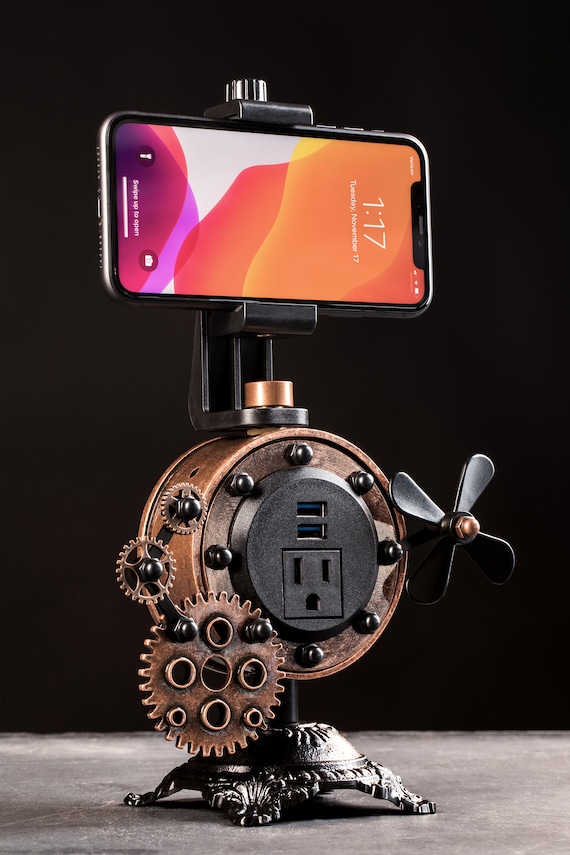The image depicts an elaborate steampunk-inspired phone stand positioned on a gray stone surface against a black background. The stand features an intricate assembly of brass gears and cranks, giving it a distinctive cyberpunk aesthetic. Atop the stand, a smartphone, likely an iPhone, is held in a sideways orientation. The phone screen shows the time as 1:17 on Tuesday, November 17th, with a vibrant background featuring hues of yellow, orange, pink, and purple, and a swipe-up to unlock prompt. The stand includes functional components such as a small fan on the right and a central copper gear that houses a traditional three-prong outlet and two USB ports. The base of the stand is crafted from dark, cast-iron with clawfoot elements reminiscent of antique designs, contrasting with the modern features and adding to its Frankenstein-like, whimsical steampunk appearance.